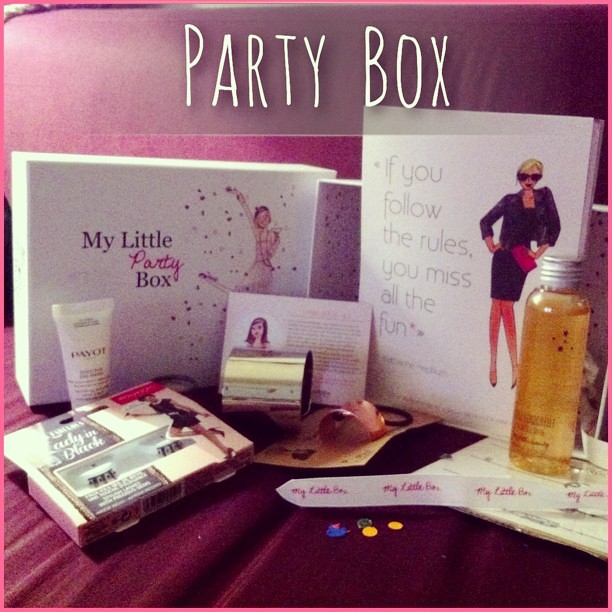This color photograph depicts a meticulously arranged display of makeup and personal care items, all elegantly positioned on a maroon cloth backdrop. At the top, bold text reads "Party Box," and on the left side, the words "My Little Party Box" are prominently displayed. The setup includes a variety of items: a white tube of cream, a neatly packaged set of false eyelashes, a shiny silver cup situated centrally, and a container of golden liquid—likely shower gel or lotion—with a silver screw-on top.

Adding to the aesthetic, a poster on the right side declares, "If you follow the rules, you miss all the fun," encapsulating the playful spirit of the arrangement. The items are a vivid mix of colors including light brown, gold, pink, dark blue, light pink, purple, yellow, and fuchsia, all carefully arranged yet seemingly spread out randomly. The photograph is taken straight on, capturing the entire collection of products. Additional decorative elements such as little flower petals enhance the overall festive look, suggesting it's an imaginative gift box, potentially ordered online and delivered as a delightful surprise.